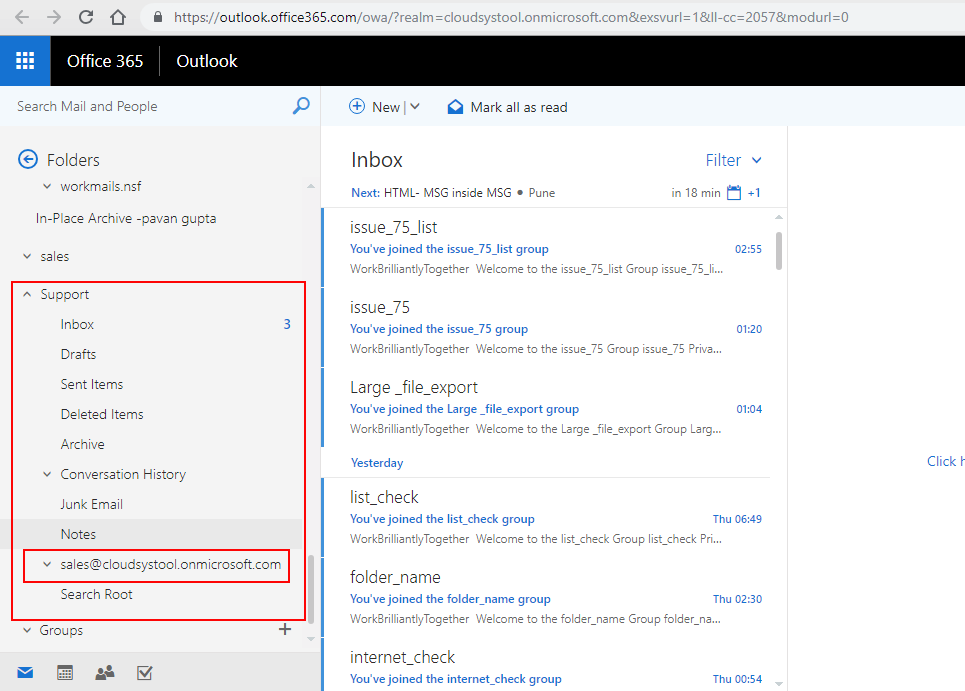Here is an enhanced and detailed caption based on the provided information:

---

This image showcases the Microsoft Office Online interface for Outlook, accessible via outlook.office365.com with an extended Realm URL. The top toolbar features essential navigation tools, including back and forward arrows, a refresh button, and a home icon. A prominent blue icon with nine white dots is visible, indicating the app launcher, beside the labels "Office 365" and "Outlook" in white font on a black background.

The user interface includes a blue search bar labeled "Search Mail and People," along with options to create new mail or mark all items as read. The left sidebar displays various folders and categories, including:
- **Folders**:
  - Workmails.nsf
  - In Place Archive
  - Pavan Gupta
  - Sales

A red rectangle outlines a specific section detailing:
- Support
- Inbox
- Drafts
- Sent Items
- Deleted Items
- Archive
- Conversation History
- Junk Mail
- Notes
- Sales and Clouds
- Systool.onmicrosoft.com
- Search Root

Within this red-outlined section, another red rectangle highlights the "Sales and Cloud Systool.onmicrosoft.com" folder. To the right, the interface shows various groups that the user has joined, categorized under "Groups" beneath the outlined sections.